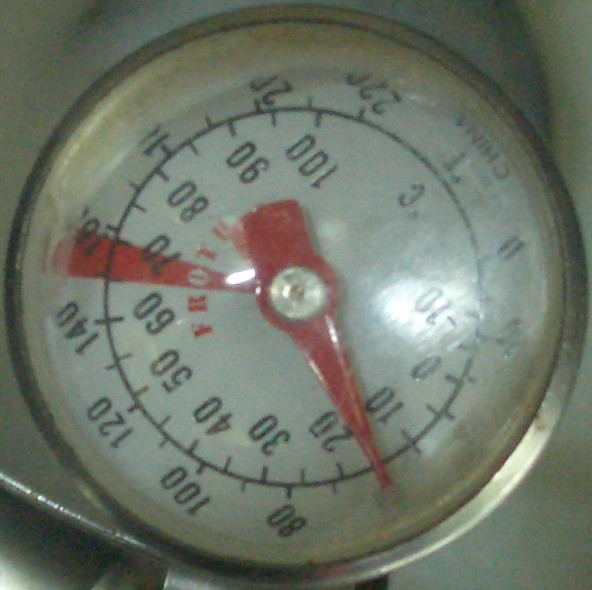A detailed close-up shot features a pressure gauge. The gauge's face is white with black numerical indicators and line increments, marked clearly for precise readings. A prominently displayed red arrow, affixed by a central circular silver screw, serves as the indicator needle. The needle points to a position between the numbers 10 and 20, indicating a measurement of approximately 15 units. The upper right corner of the gauge face bears the text "China," while the perimeter of the gauge face is inscribed with red text reading "Froth." The entire gauge is protected by a clear glass cover, which is bordered by a sleek silver metal frame, adding a polished finish to the instrument's design.